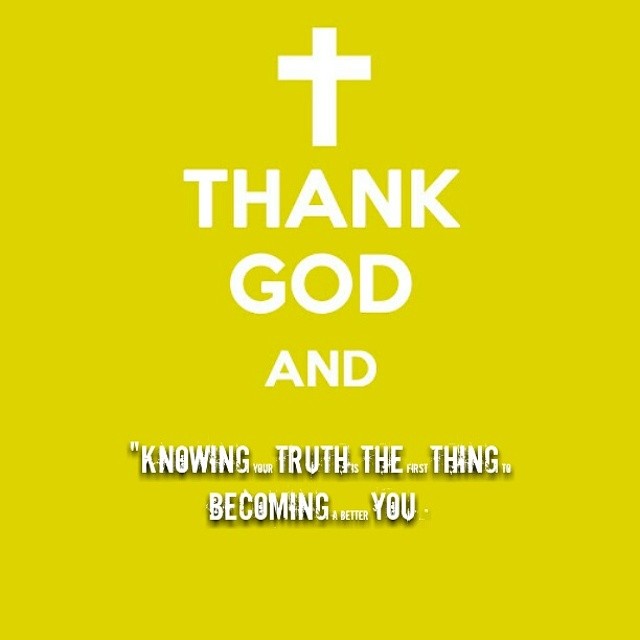The image features a prominent white cross at the top center against a bright yellow background. Below the cross, large white text declares "THANK GOD." Beneath this, another line in white text reads: "KNOWING YOUR TRUTH IS THE FIRST THING TO BECOMING A BETTER YOU." The phrase employs varying text sizes for emphasis: "KNOWING," "TRUTH," "THING," "BECOMING," and "YOU" are large, while "YOUR," "IS," "THE," "FIRST," "TO," "A," and "BETTER" are much smaller. The entire composition, with its capitalized words and striking color contrast, creates a bold and somewhat chaotic visual message on the yellow background.